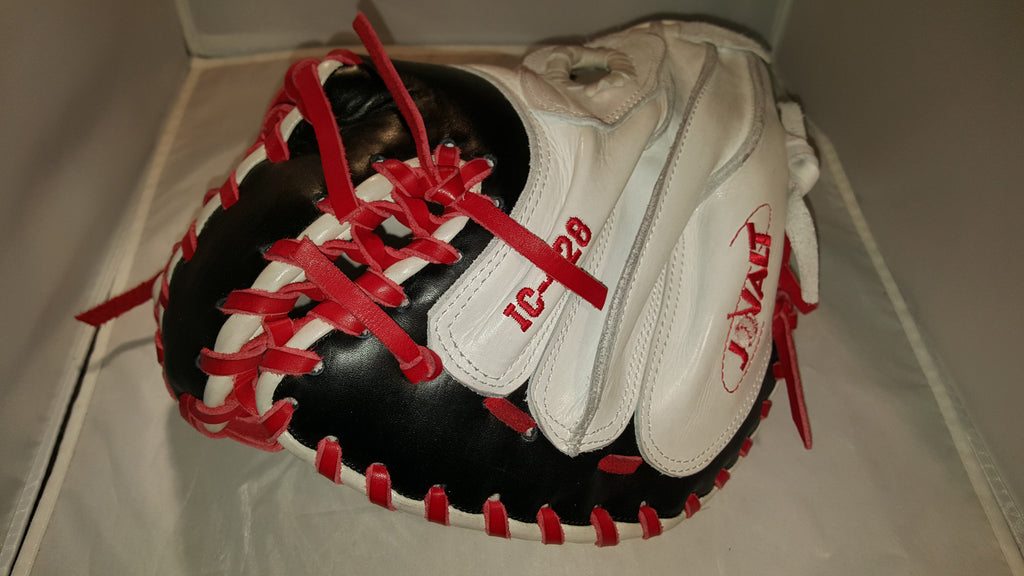The photograph features a baseball catcher's mitt, predominantly white with black on the inside and red accents throughout. The red stitching and lacing hold the mitt together, and there is red embroidery displaying the letters "IC-28" and the word "JVALT." A small baseball is also embroidered on the mitt. The glove is positioned facing downward, with its back and the red-lettered inscriptions clearly visible. It is placed inside a white, fabric storage box, enhancing the contrast of its tricolored design against the pristine background. The setting appears meticulously arranged to highlight the details of the glove within the confines of the box.